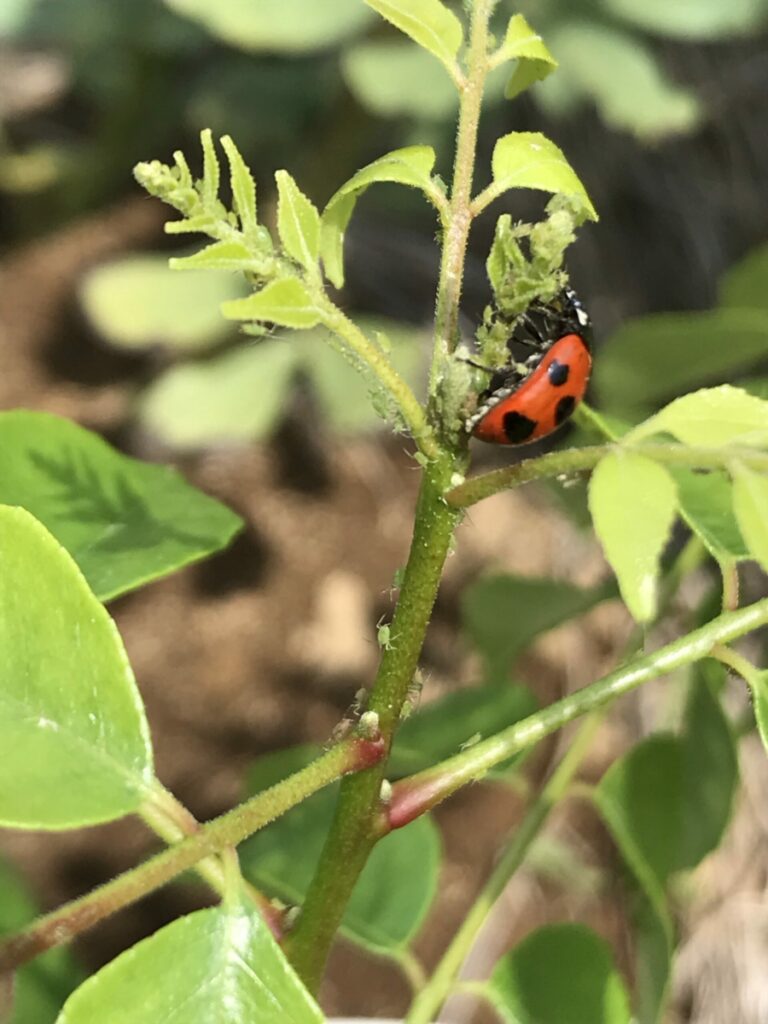In this vivid close-up photograph, a red ladybug with distinct black spots clings to the tip of a spiny, vine-like green plant. The ladybug appears to be munching on the freshly blossoming leaves. The plant, which resembles a tomato plant, stretches up with one main stem and several offshoots. The background is an artful blur of earthy browns, lush greens, and occasional hints of black, creating a bouquet effect that highlights the plant and the ladybug in sharp detail. It's a bright, clear day, allowing for an intricate view of the spiny surface of the plant and the vibrant colors of the scene. The image encapsulates the vivid interaction of the ladybug and its leafy perch against a softly shadowed, natural backdrop.